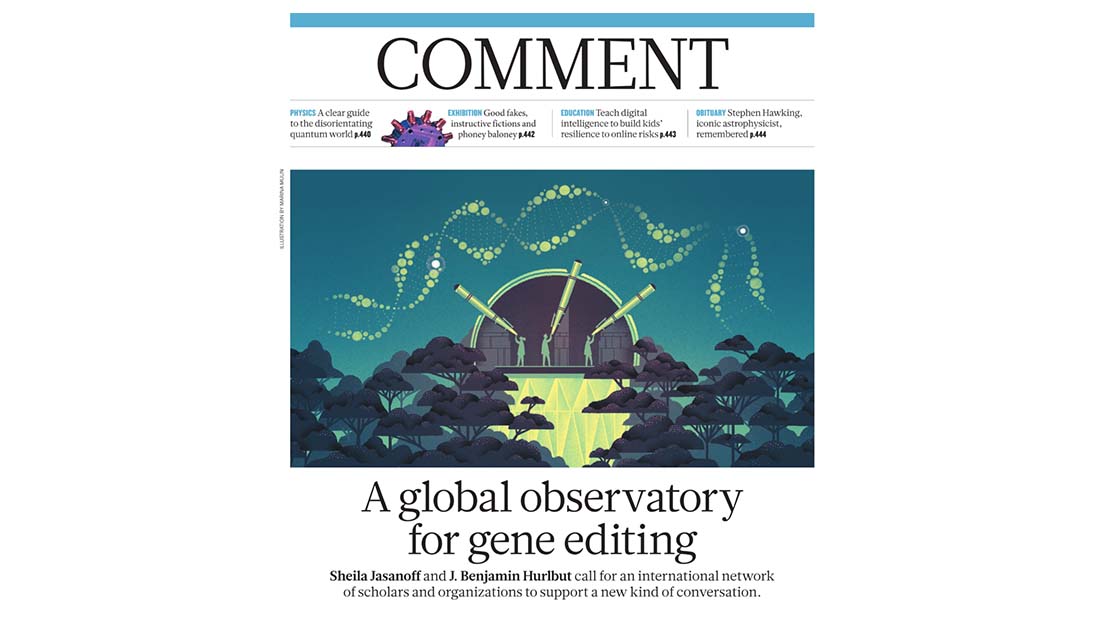This image, styled like a magazine article, appears to be an advertisement or announcement. At the very top is a light blue bar running across the width of the image. Below this bar, in large, bold black font, is the word "Comment". 

Underneath this heading are four distinct blurbs, each with accompanying page numbers:
1. "Physics: A Clear Guide to the Disorienting Quantum World" - Page 440.
2. "Exhibition: Good Fakes, Instructive Fictions, and Phony Baloney" - Page 442.
3. "Education: Teach Digital Intelligence to Build Kids' Resilience to Online Risks" - Page 443.
4. "Obituary: Stephen Hawking, Iconic Astrophysicist Remembered" - Page 444.

Dominating the visual space is a large, detailed image of an observatory, viewed from the front. The observatory is surrounded by trees, and in front of it are three individuals peering through large telescopes. These telescopes are configured in an arch shape above the round observatory, spiraling in a manner reminiscent of a DNA helix.

At the bottom, another title reads: "A Global Observatory for Gene Editing."